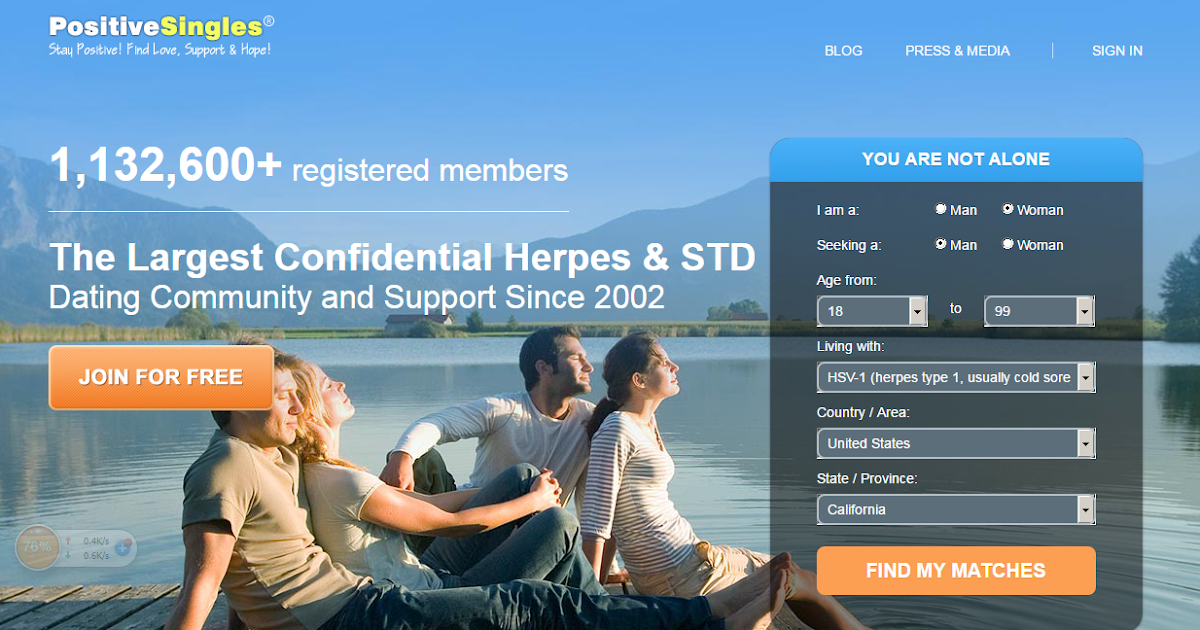This is a detailed description of a webpage from the business called Positive Singles:

The webpage prominently features the Positive Singles logo in the upper left-hand corner. The logo combines the words "Positive Singles" into one, with "Positive" in bold white text and "Singles" in bold yellow text. Below the logo, a motivational tagline in a thin, casual white font reads, "Stay Positive! Love, Support, and Hope!"

On the far right side of the header, navigation options are displayed in white text: "Blog," "Press and Media," and "Sign In." 

Below this header, off to the left, bold white text announces that there are "1,132,600+ registered members." A thin white line separates this figure from a subsequent claim, in bold white text, stating, "The Largest Confidential Herpes and STD Dating Community and Support Since 2002"—with "Dating Community and Support Since 2002" in regular, non-bold white text. 

Further down, a prominent orange button invites users to "Join for Free."

To the right of this button, a semi-transparent black box overlays the background image. The top of this box is accentuated by a bright blue banner that declares, "You Are Not Alone" in white text. Below, there are selectable options: users can specify, "I am a man or woman seeking a man or woman," filter age from 18 up to a maximum of 99, choose the condition they are living with from a drop-down menu starting with "HSV-1, Herpes Type 1, usually cold sore," and select their country or area. In the current view, "United States" and "California" are displayed as the chosen location. At the bottom of this section, an orange box with white text urges users to "Find My Matches."

The webpage's background is dominated by a serene, sunlit image of two couples sitting on a dock by a lake. The women are lifting their faces towards the sun, appearing to soak in its warmth, while the men have their eyes closed, basking in relaxation. This picturesque scene is set against a backdrop of tranquil mountains and a placid, glass-like lake under a clear, blue sky.